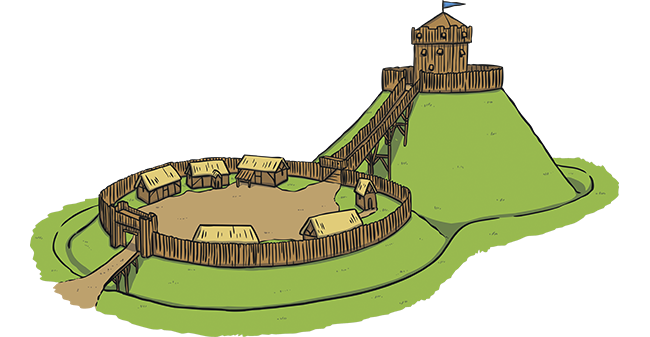The image is a brightly colored cartoon illustration of a medieval Motte and Bailey. In the foreground, a brown pathway winds from the bottom left corner towards the entrance of a wooden palisade. This palisade, circular in shape, encloses a small village with five straw-roofed wooden buildings arranged around a dirt courtyard. The village occupies a lower, broader hill and is surrounded by lush green grass. Around both hills, a moat filled with water is visible.

Towards the back of the village, a wooden bridge ascends to a taller hill in the background. This hill appears to have its top flattened, and atop it stands a singular wooden tower adorned with a blue flag. The tower is enclosed by another palisade with closely spaced wooden slats, reinforcing its defensive nature. This secondary structure likely serves as the castle or fortress keep. The vantage point of the illustration is from a distance, giving a comprehensive view of the hill fort's layout and the interconnectedness of the two hills.